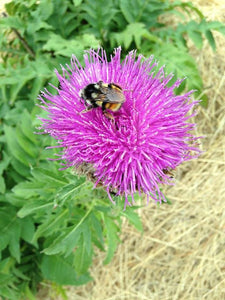This is a detailed, close-up vertical image of a large, vibrant purple flower with delicate thin petals that have white tips, forming a distinctive, spherical shape. A yellow and black bumblebee, characterized by its horizontal, rectangular body shape and slightly rounded end, is perched atop the flower. The bee's wings are a light brownish-yellow, lying flat on its back. The photo is taken from an overhead angle, highlighting not only the bee's detailed search for pollen but also the flower's green leaves and stems. The background features a mix of green shrubs and noticeably dried blades of grass, providing a contrasting backdrop to the colorful focal point.